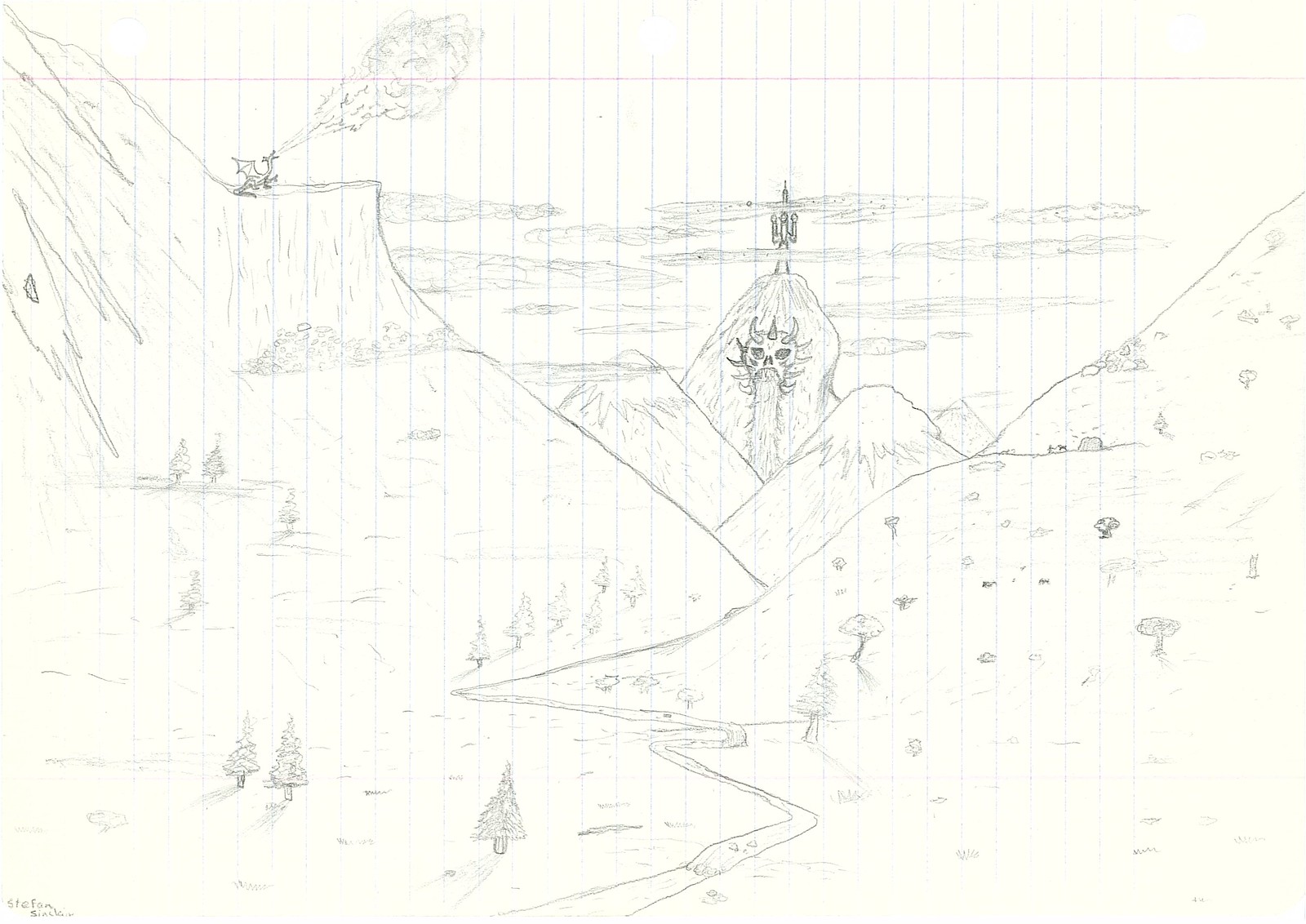This is a highly detailed hand-drawn image in black or gray pencil on a piece of wide-ruled notebook paper that has been rotated horizontally. The paper features the familiar blue horizontal lines and the red margin line, now running along the top of the image, as well as hole punches along what is now the left side. The scene depicts a dramatic mountainous landscape with multiple snow-capped peaks flanking a central valley through which a winding river flows. The mountains on the left and right edges frame the composition, with the central mountain being particularly prominent and pointed at the top. This mountain intriguingly features a monstrous skull with spikes, from which a liquid is spewing out, resembling water flowing from its mouth. On top of this central mountain, there appears to be a structure that might be a castle with towers. A significant fire-breathing dragon is perched atop a flattened ledge on the left mountain, emitting a plume of smoke or fire that's disproportionately large compared to the dragon itself. Scattered around the valley are various trees, resembling pines or Christmas trees. Additional elements include clouds floating in the sky and a hand-written signature located in the bottom left corner of the page, reading "Stéphane Sinclair." The vivid details and the fantastical elements combine to create a captivating and imaginative landscape.